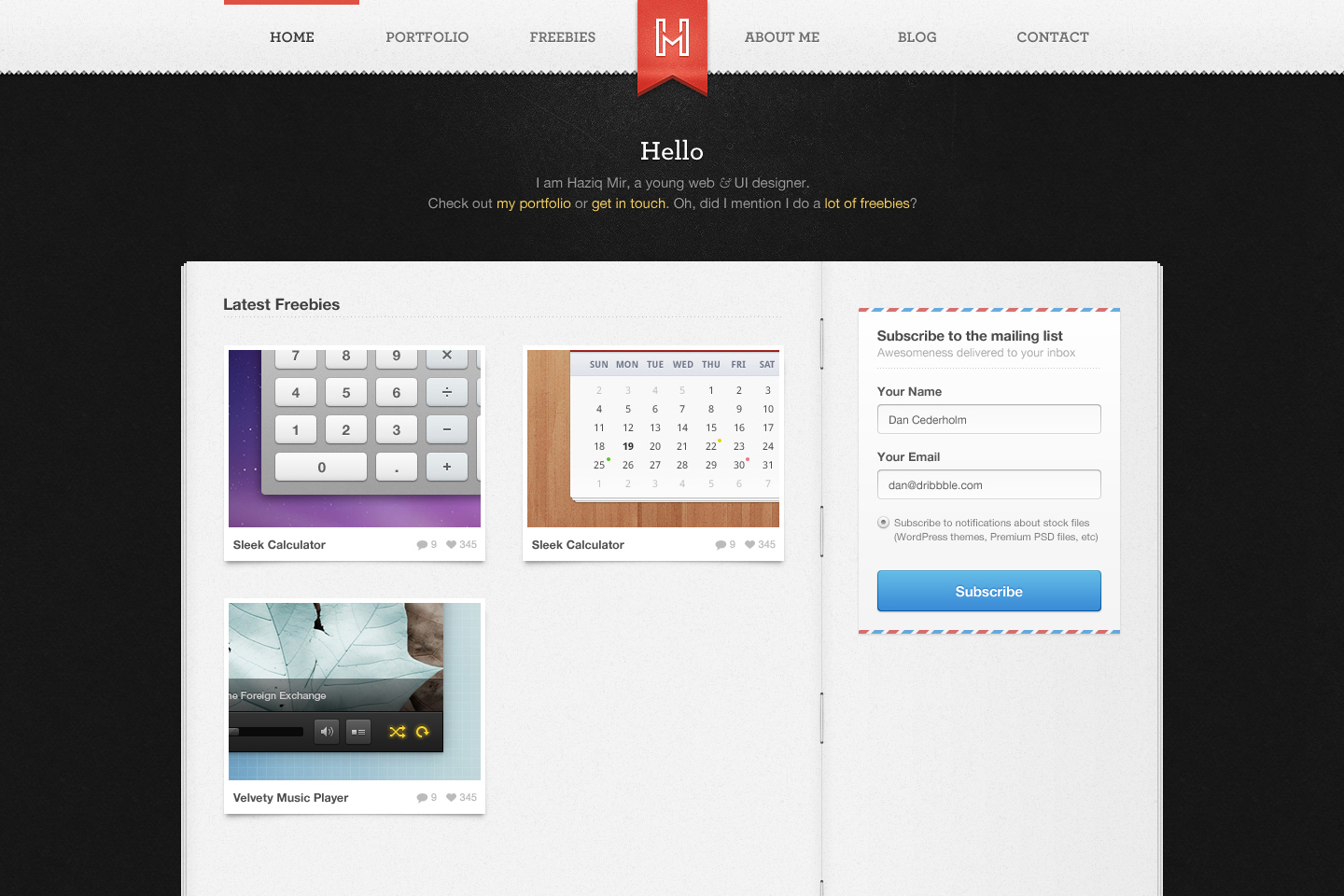This screenshot captures a detailed visual of a web designer's portfolio website. The top section showcases a navigation bar set against a white background, featuring tabs labeled Home, Portfolio, Freebies, About Me, Blog, and Contact, aligned from left to right. Centrally placed between Freebies and About Me is the website's logo, illustrated in a unique orange ribbon design that descends from the top of the screen. The logo itself resembles the letter 'H' with a distinctive bend in the middle, forming an 'M' shape.

The highlighted 'Home' tab indicates the current page viewed. Above the navigation bar, a black banner introduces Hazig Mir, highlighting his profession as a young web UI designer with an invitation to explore his portfolio and connect with him. The introductory text reads, "Hello, I am Hazig Mir, a young web UI designer. Check out my portfolio and get in touch, or get in touch. Oh, did I mention I do a lot of freebies?"

Below this introduction, the section titled 'Latest Freebies' displays various design assets created by Hazig Mir, including two sleek calculators, a sleek calendar, and a Velvety Music Player. These showcased items reflect his expertise and offer potential clients a chance to test and review his work, encouraging them to reach out for possible collaboration.